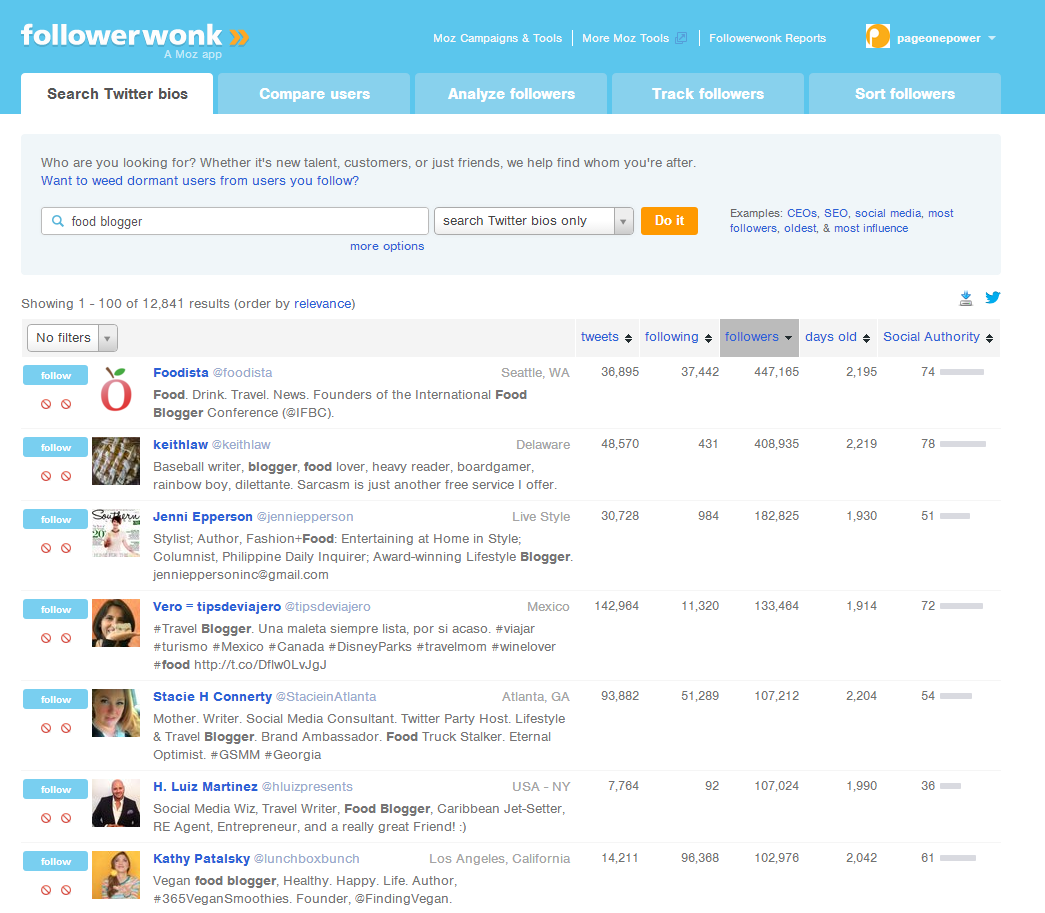This screenshot captures a page from FollowerWonk, a tool by Moz. At the top, there is a vibrant blue banner spanning the width of the page with white text that reads "FollowerWonk, a Moz app." To the right, it displays "Moz campaign and tools," "more Moz tools," and "FollowerWonk Nepeta," concluding with "Page One Power."

Just beneath the banner, there is a stark white rectangle featuring the black text "Search Twitter Bios." Below this, four lighter blue rectangles contain the options "Compare Users," "Analyze Followers," "Track Followers," and "Sort Followers."

Further down, another rectangular section poses the question, "Who are you looking for?" and offers assistance in finding new talent, customers, or friends, and in identifying dormant users. A search bar containing the text "Food Blogger" is positioned next to a drop-down menu labeled "Search Twitter Bios Only," followed by a prominent orange rectangle with the white command "Do It."

Examples such as "CEOs," "SEOs," "social media," "most followers," "oldest," and "most influence" are listed below. The section also displays a summary: "Showing 1-100 of 12,841 results, ordered by relevance," followed by a statement "No Filters" and a display of individual profiles, starting with "Foodista."

The ensuing list features user profiles with their respective statistics like tweet count, followings, followers, account age, and social authority. The visible profiles include "Keith Law," "Jenny Epperson," "Vero Tips DeVivero," "Stacey H. Connerty," "H. Luis Martinez," and "Kathy Patowski."